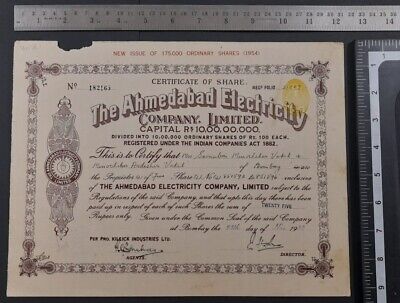This detailed photograph features an old, worn stock certificate from The Ahmedabad Electricity Company Limited, prominently centered against a black background. At the very top of the certificate, in bold red letters, it states "New Issue of 175,000 Original Shares, 1954." Beneath that, the certificate is titled "Certificate of Share," with additional text indicating "Capital R, 10 million" and cursive script certifying authenticity. The stock certificate is bordered by two metal rulers: one ruler horizontally positioned above the certificate measuring up to 12 inches, indicating its width, and another vertically along the right side, measuring up to 9 inches to show its height. The colors in the image include shades of yellow, black, gray, red, and silver, adding to the vintage and detailed presentation of the historical document.